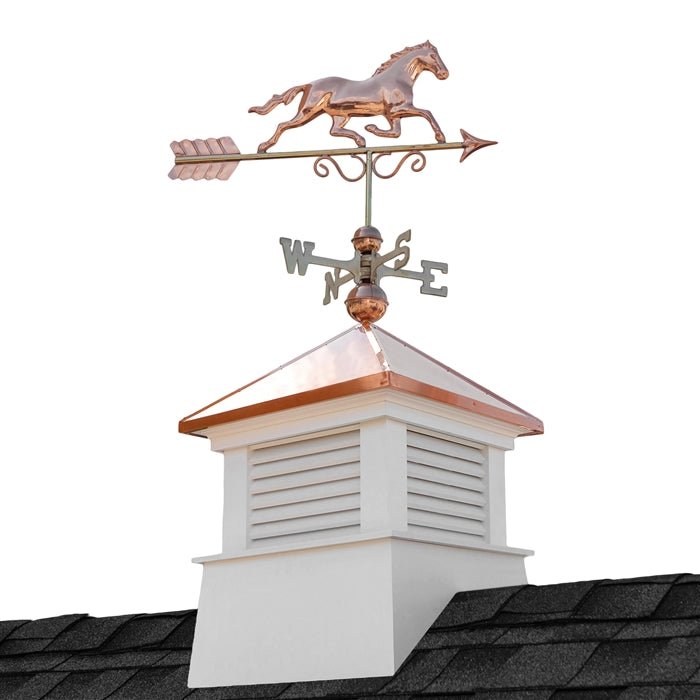This image captures a detailed view of a rooftop section covered with composition shingles. In the center of the image, a white-painted cupola with distinctive louvered slats can be seen. The cupola features a hipped roof made of copper, which is topped by an ornate weather vane. The weather vane includes directional signs (N, S, E, W) arranged around a central post, with spherical accents placed both above and below the directional indicators. Above this setup, a copper arrow points to the right, anchored by a figure of a galloping horse crafted from the same copper material. The backdrop of the image is a blank white screen, enhancing the contrast and details of the structures. The meticulous design and polished appearance hint at either a modern build, a newly installed feature, or a digitally enhanced representation.